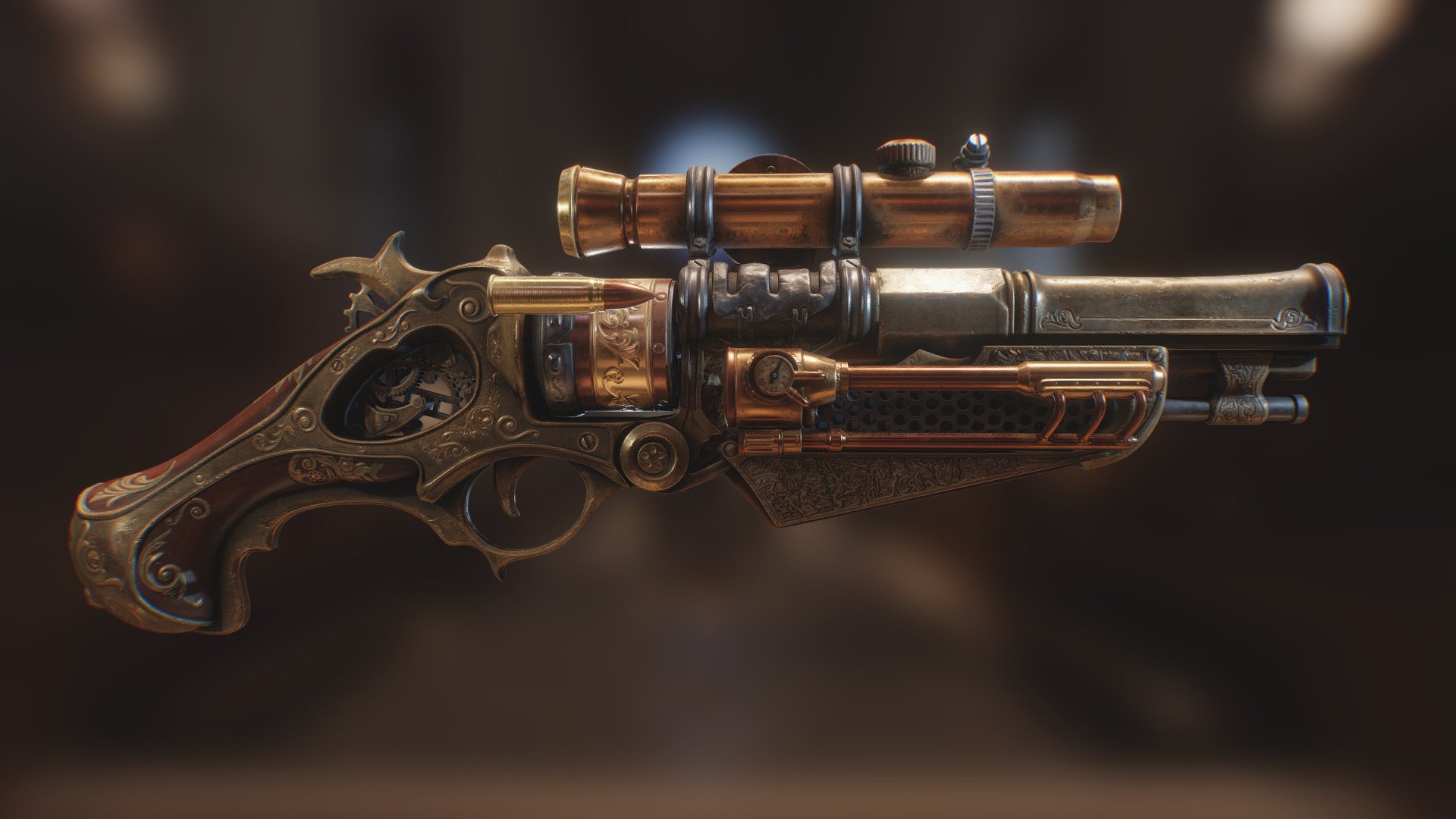This image, likely AI-generated, depicts an intricately designed steampunk-style handgun that combines elements of futuristic and vintage aesthetics. The gun features an ornate handle made of wood with scrolling metal engravings in faded brass or dark gold, giving it a worn, artistic look. The silver barrel appears slightly dirty and used, adorned with an elaborate brass decoration that includes a small pressure gauge with numbers on it. Attached to the top of the barrel is a copper scope, adding to the gun's unique character. The background of the image is blurred in shades of gray, black, and off-white, emphasizing the intricate details and craftsmanship of the weapon.